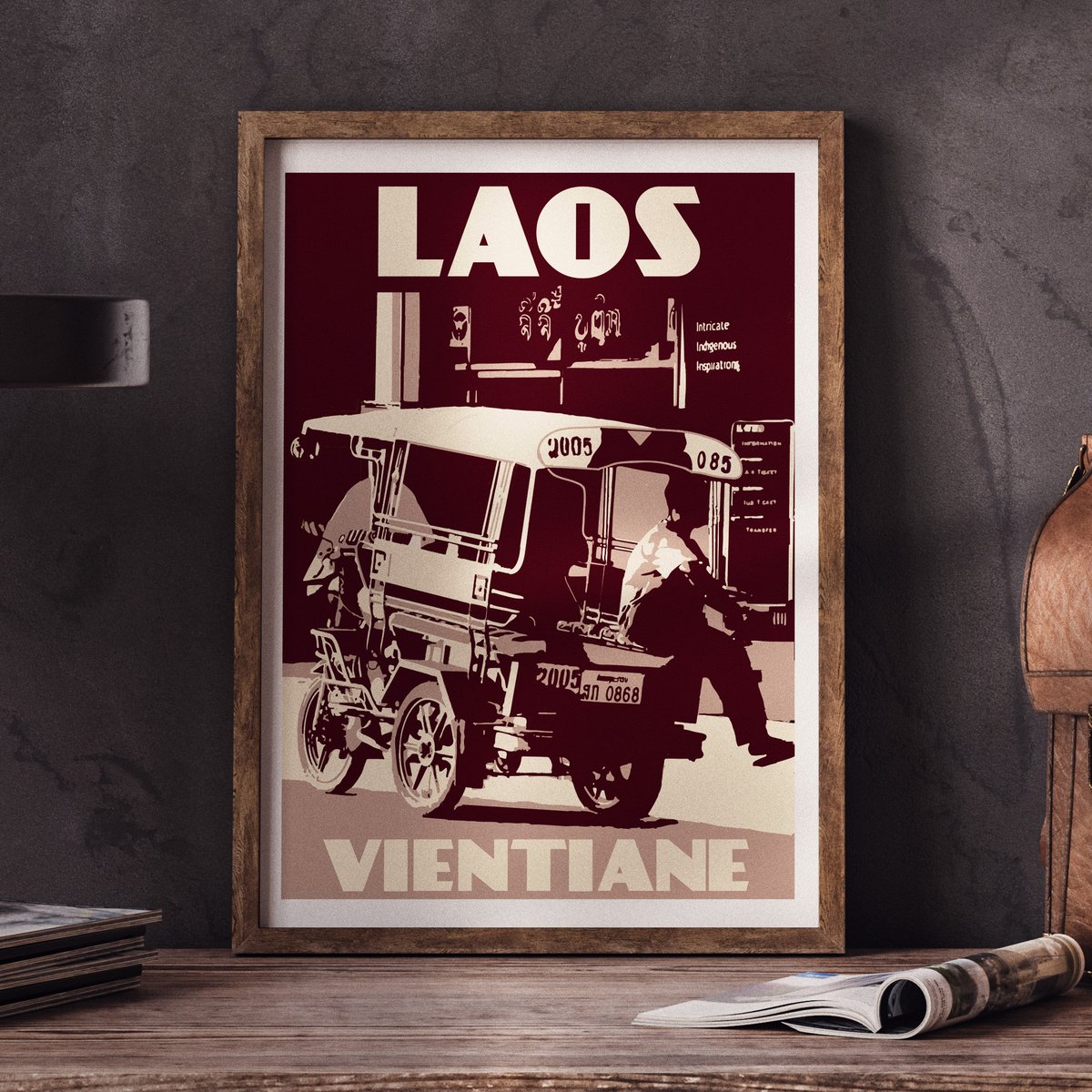This is an intricately detailed digital creation made to resemble an old photograph, framed and set against a gray wall with darker streaks. The centerpiece of the image is a dark burgundy or maroon poster with cream and brown highlights. At the top of the poster, "LAOS" is prominently displayed in white capital letters. Below this, there is an old-fashioned, small motorized vehicle, possibly a taxi-like mobile, featuring a man sitting in its open back with his feet hanging out. Both sides of the back of the vehicle display the numbers "2005" and "085." The lower left corner of the poster repeats "2005," and there's a license plate marked "AN 0868." At the very bottom, "VIENTIANE" is written in cream letters. The entire scene is enclosed within a wooden frame resting on a wooden table. Surrounding the framed poster, there is an out-of-focus open magazine on the bottom right, a partially visible brown messenger bag on the right side, several stacks of magazines or books on the lower left, and an unclear cylindrical object in the upper left. The overall composition creates a nostalgic ambiance with vintage tones and textures.